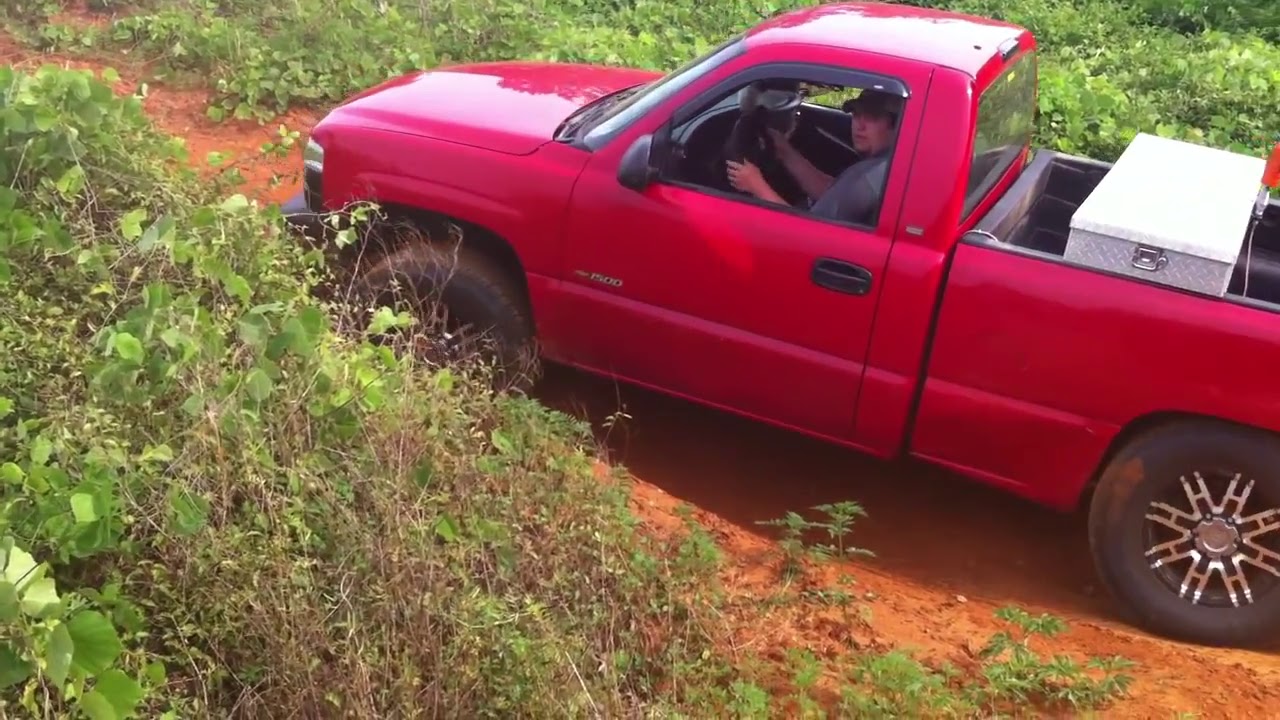The photograph captures a bright cherry red mini truck navigating a narrow, unmetalled, brown dirt path amidst lush greenery. The truck's driver, donning a dark gray t-shirt and a matching baseball cap, has his hands on the steering wheel and is glancing towards the viewers from his dark-interior vehicle. The truck features black door handles and shiny silver wheels. In the bed of the mini truck, there is a large, metallic, white trunk with silver handles, alongside an orange-bristle brush. The entire scene is set outdoors, showcasing the contrast between the brown dirt path and the vibrant green plants surrounding it.